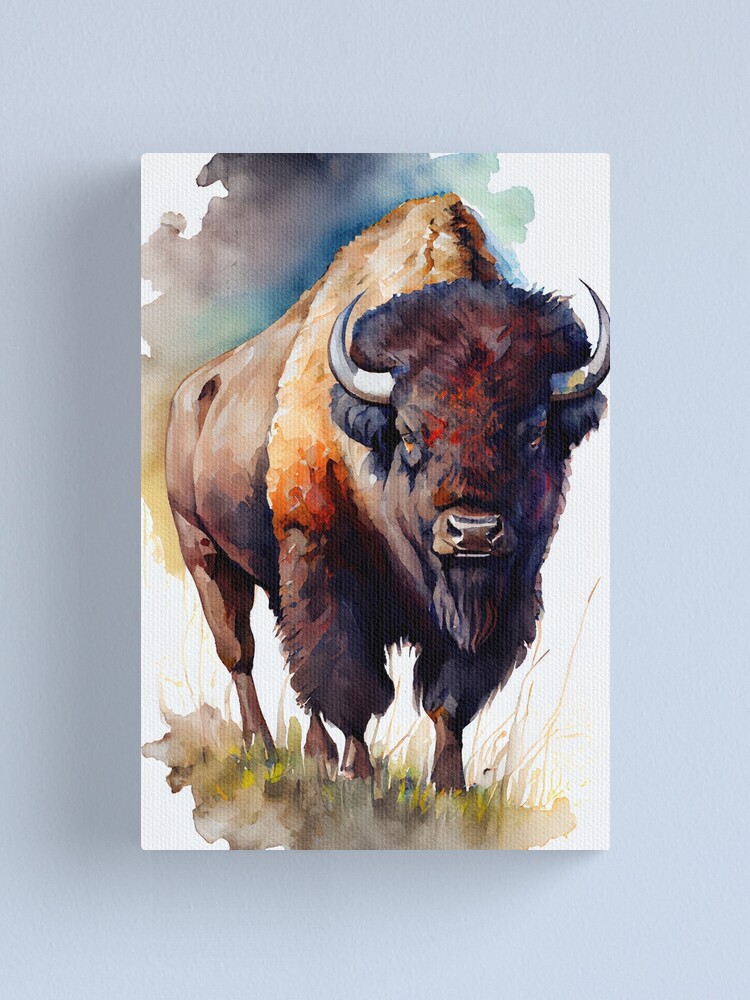This image is a detailed watercolor print of a buffalo, with the painting set against a periwinkle blue wall. The buffalo is centered in the composition, facing forward, allowing a view of part of its body extending left. The light seems to be hitting it from the left side, casting a gentle illumination over its figure. The buffalo is illustrated with dark reddish-brown fur on its face and front legs, complemented by a lighter beige on its prominent hump, and extending to a dark brown across the rest of its body. Small, sharp white horns curve upward from each side of its head, and its wide nose and the reddish-black fur on its head add to its detailed expression.

The background of the painting is a white expanse accentuated by watercolor splashes. These splashes transition from yellow to green to blue, eventually deepening into navy, suggesting a dynamic sky, possibly at sunrise. Below the buffalo, a muddy brown base blends into vibrant green and yellow plant growth with hints of beige and some weeds emerging from the watercolor ground. The eyes of the buffalo, detailed in yellow and black, stare directly at the viewer, creating a striking and vivid portrayal.